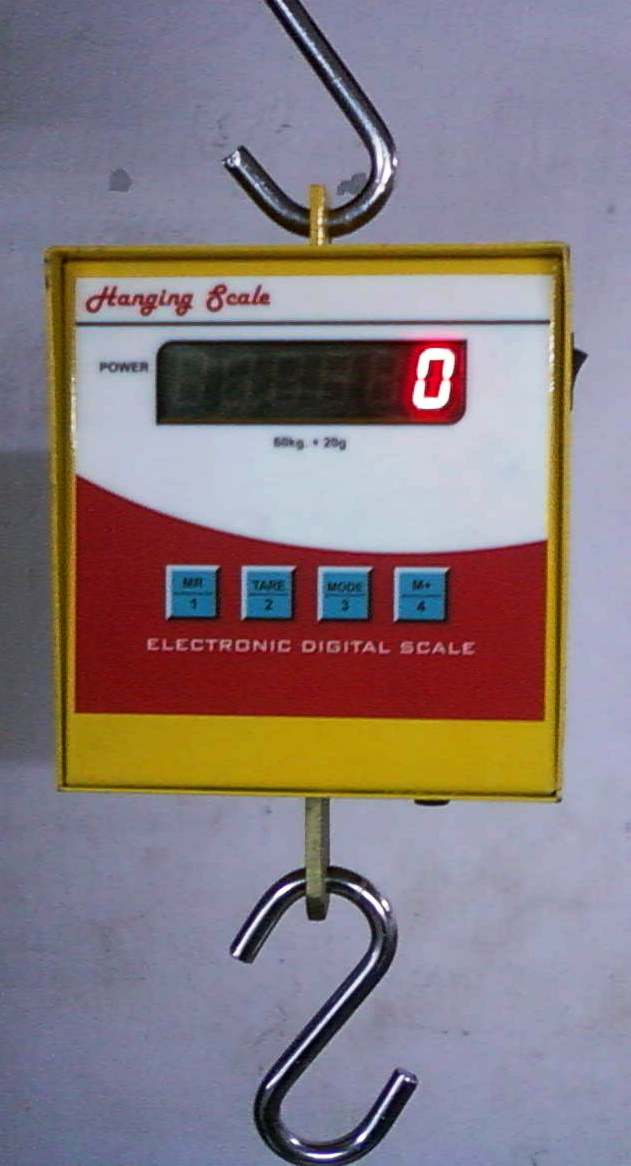This highly detailed photograph features an electronic digital hanging scale against a light bluish-purplish background in portrait orientation. The scale, predominantly yellow with red and white accents, hangs from a set of metal hooks. At the very top, a bottom part of a hook is visible, connected to a small gold ring. Below, there's a yellow frame of the scale with a white label on the top half and a red label on the bottom half. The top left corner of the scale features the words "Hanging Scale" in red cursive, possibly indicating its function or brand.

A prominent digital screen displays a red "0", suggesting the scale is currently not measuring any weight. Beneath the screen, there are blue buttons labeled "Tare," "Mode," "M+," and numbered 1 to 4. Additionally, text reading "Electronic Digital Scale" is inscribed in white. Visible at the very bottom of the image is a reversed S-shaped metal hook attached to the yellow-framed scale, with an S-hook connecting at the bottom. The entire setup appears designed to measure weight efficiently, with all functionalities clearly indicated by various color-coded labels and digital indicators.